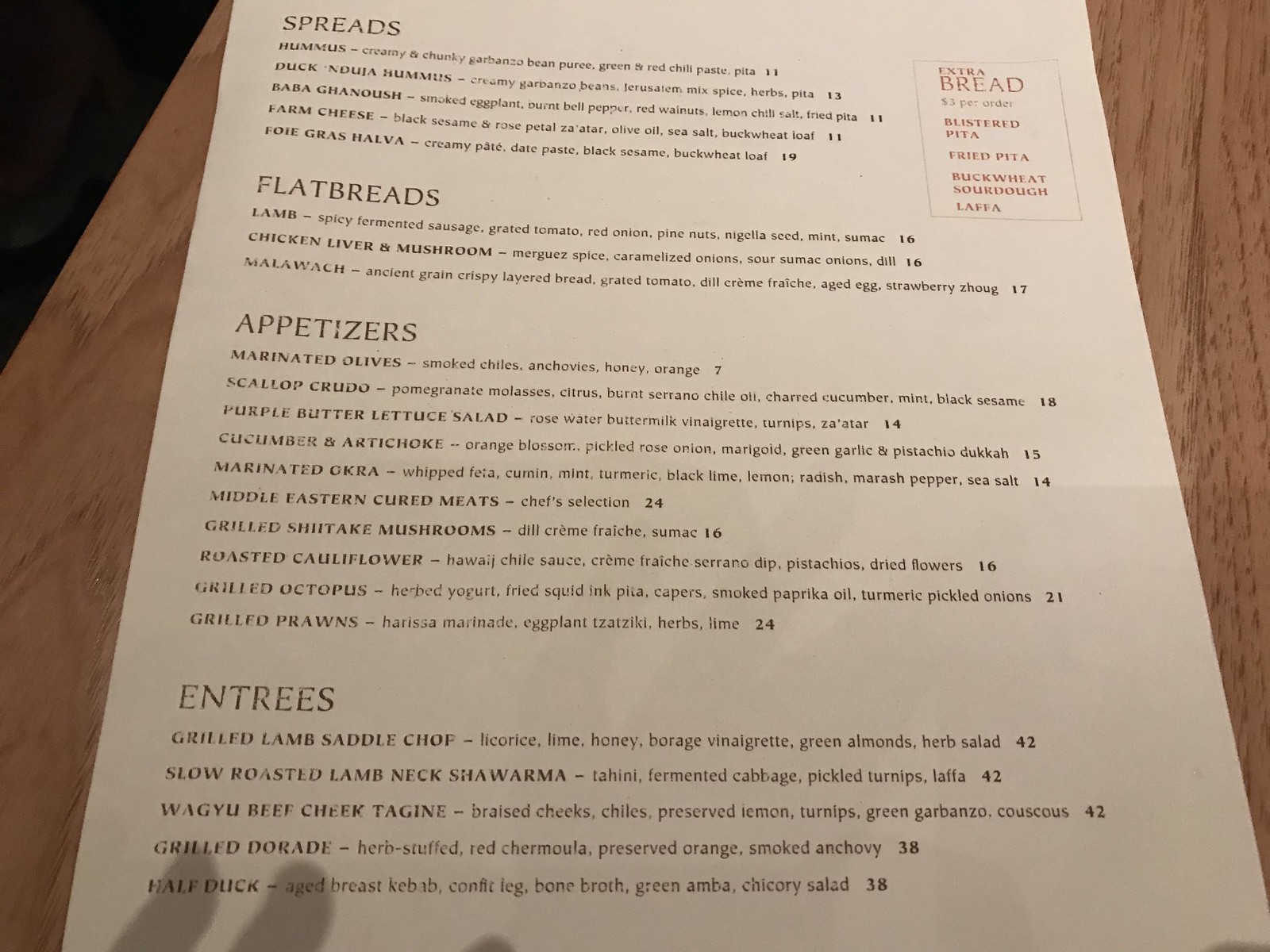The image depicts a menu printed on plain white paper, resting on a table with a laminate wood effect. The menu features black text, with main sections titled in bold capital letters: SPREADS, FLATBREADS, APPETIZERS, and ENTREES. In the top right corner, there is a red text box that reads: "Extra bread, $3 per order," listing options such as blistered pita, fried pita, buckwheat sourdough, and laffa.

Under the SPREADS section, prices range from $11 to $19. Options include:
- Hummus ($11)
- Duck and Judah Hummus ($13)
- Baba Ghanoush ($11)
- Farm Cheese ($11)
- Foie Gras Halva ($19)

For FLATBREADS, prices are either $16 or $17:
- Lamb ($16)
- Chicken, Liver, and Mushroom ($16)
- Malawak ($17)

The APPETIZERS section lists items ranging from $7 to $24:
- Marinated Olives ($7)
- Middle Eastern Cured Meats ($24)
- Grilled Prawns ($24)

Lastly, the ENTREES are priced between $38 and $42, featuring:
- Grilled Lamb Saddle Chop
- Slow Roasted Lamb Mix Shawarma
- Wagyu Beef
- Grilled Dorad
- Half Duck